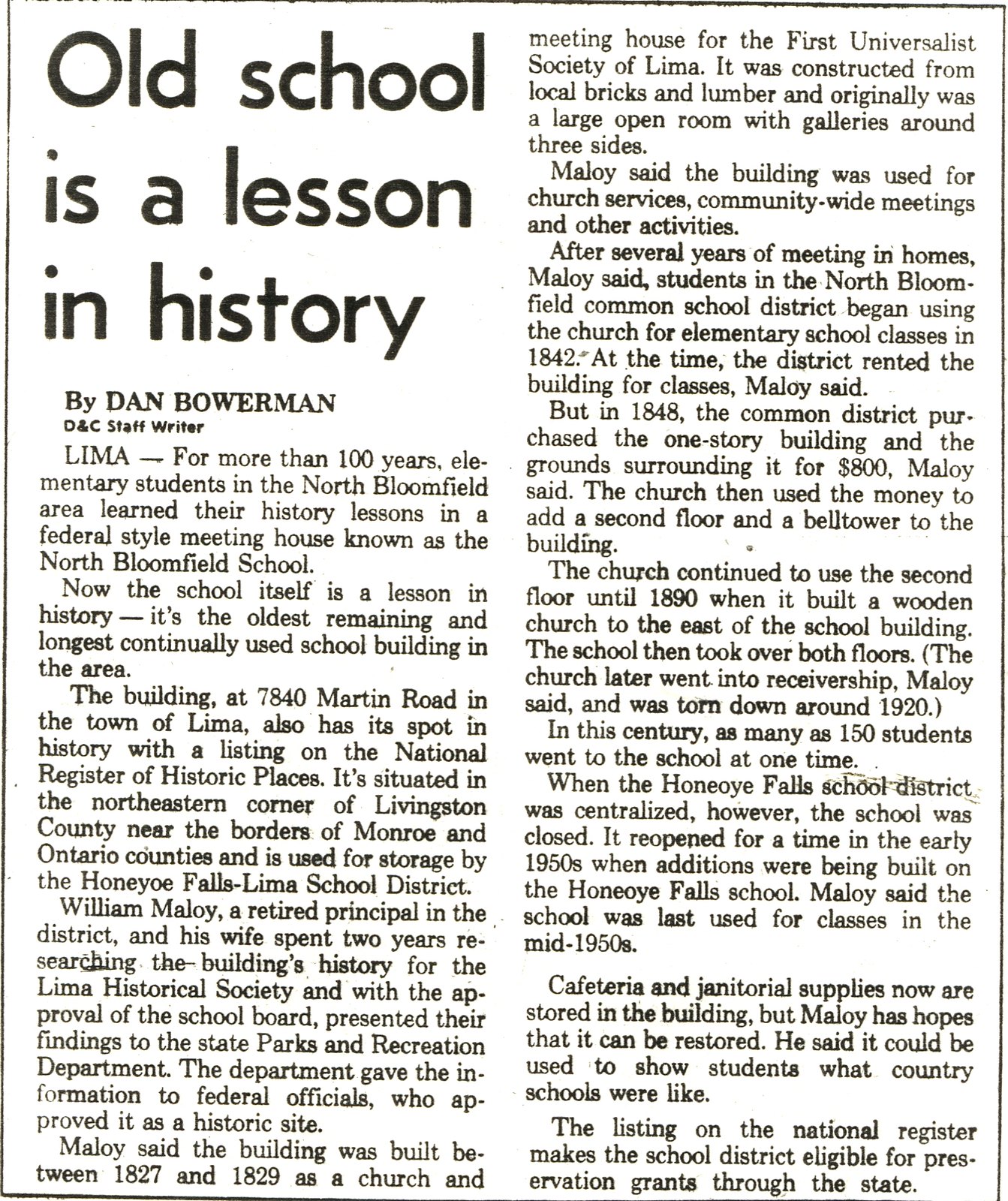This is an image of a black-and-white newspaper clipping titled "Old School is a Lesson in History" by Dan Bowerman, DNC staff writer. The article highlights the North Bloomfield School, located at 7840 Martin Road in the town of Lima. Built between 1827-1829, this federal-style meeting house served as an educational institution for over 100 years, making it the oldest remaining and longest continually used school building in the area. The building is situated in the northeastern corner of Livingston County, near the borders of Monroe and Ontario counties. It is currently used for storage by the Honeyo Falls Lima School District and holds historical significance with its listing on the National Register of Historic Places. Additionally, the article mentions retired principal William Molloy and provides further details about the school's historic status.